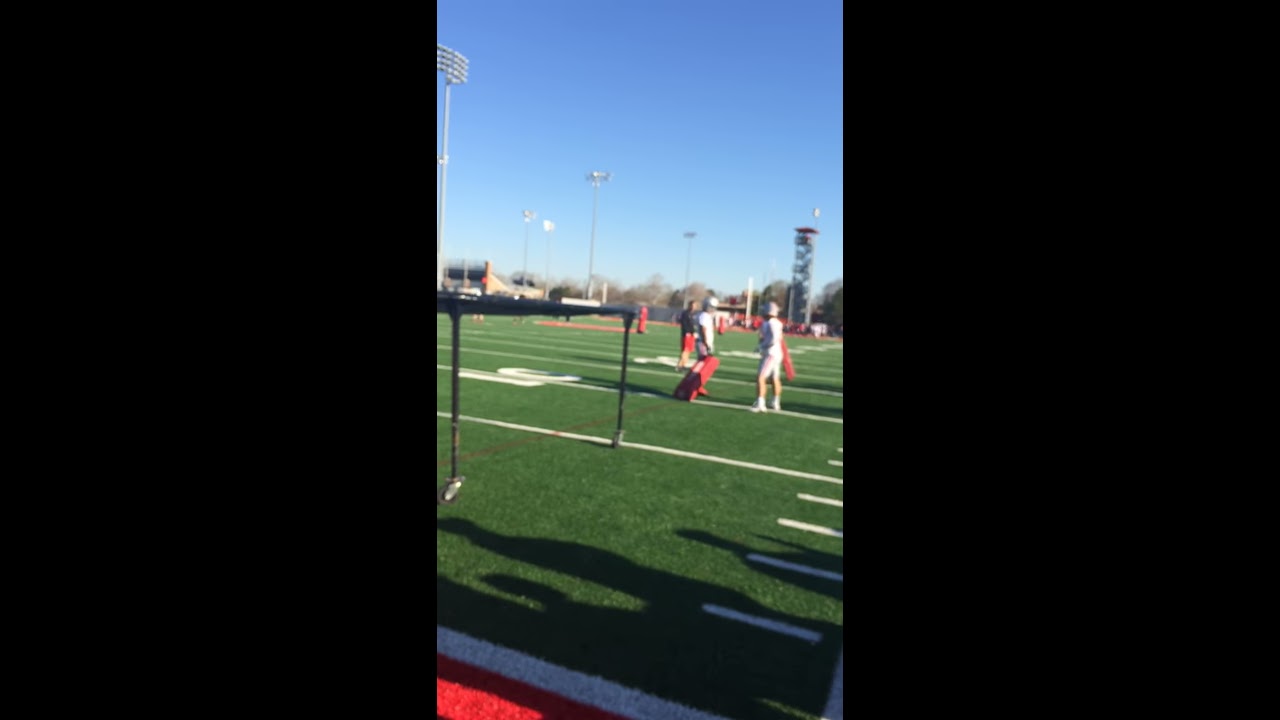This image captures a daytime scene of a football field, possibly within a stadium, with a group of people standing on the green, white-marked grass. In the foreground, close to the 10-yard line near the goal area, there are two prominently visible individuals—one appearing to be male and the other female—engaged in conversation. Nearby, football players can be seen practicing, identifiable by their helmets and light padding, rather than full game gear. The field also features a huddle area and practice dummies used for tackling drills. Surrounding elements include floodlight stands, which are unlit due to the daylight, and faint shadows cast on the field, although their sources are indistinguishable. In the background, a certain tar-like structure can be spotted, the purpose of which is unclear. Additionally, there are trees, a blue sky without clouds, and a possible watchtower, enhancing the overall serene yet dynamic ambiance of the practice session. The image, slightly blurry, encapsulates a routine day of training on the football field.